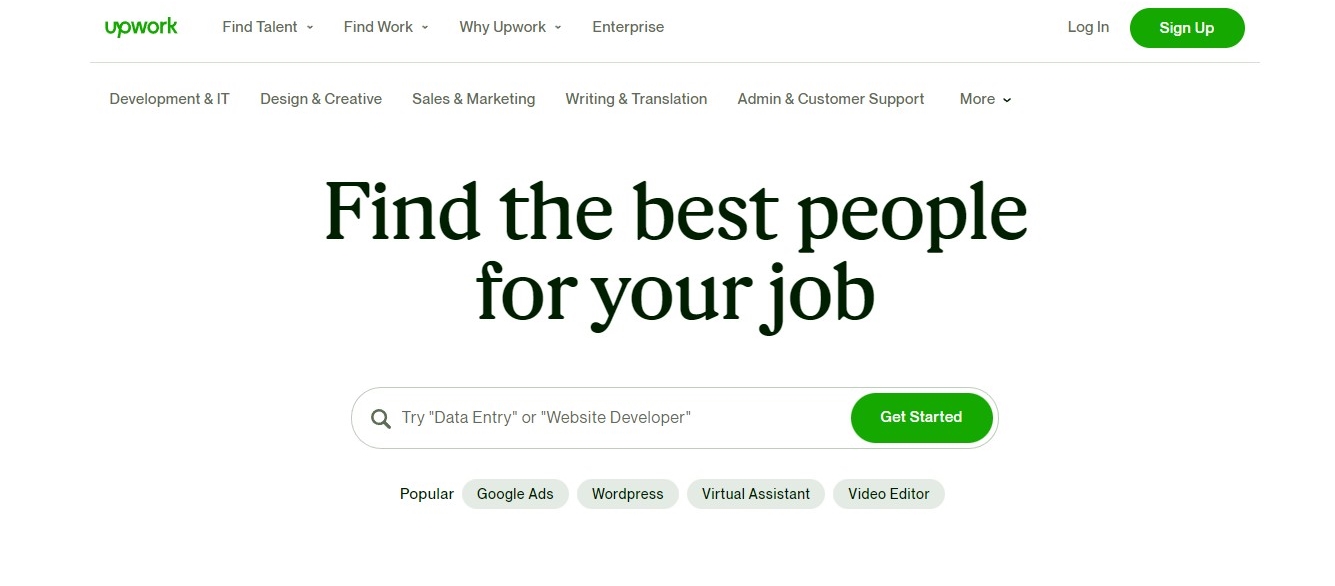The image is a left-to-right horizontal screenshot of the Upwork homepage, as it would appear on a website accessed via a smart device or computer. The background of the webpage is a clean white, blending seamlessly with the computer screen's backdrop. 

In the top left corner, the Upwork logo is prominently displayed in green. Adjacent to the logo, proceeding left to right, there are navigation links in black: "Find Talent," "Find Work," "Why Upwork," and "Enterprise." 

Towards the upper right-hand corner, there are two distinct buttons: a black "Login" button and a green "Sign Up" button with white text. 

A thin, horizontal line in gray or black separates the top navigation bar from the rest of the content below. The subsequent navigation options appear in black text and include categories such as "Development & IT," "Design & Creative," "Sales & Marketing," "Writing & Translation," "Admin & Customer Support," and more. 

Centrally located on the page is a bold, black, large-font headline stating, "Find the Best People for Your Job." Below this headline is a search bar featuring a magnifying glass icon. Inside the search bar, placeholder text reads, "Try Data Entry or Website Developer." A green button labeled "Get Started" in white text is situated next to the search bar.

At the bottom of the image, there are clickable links for popular search categories, including "Google Ads," "WordPress," "Virtual Assistant," and "Video Editor."